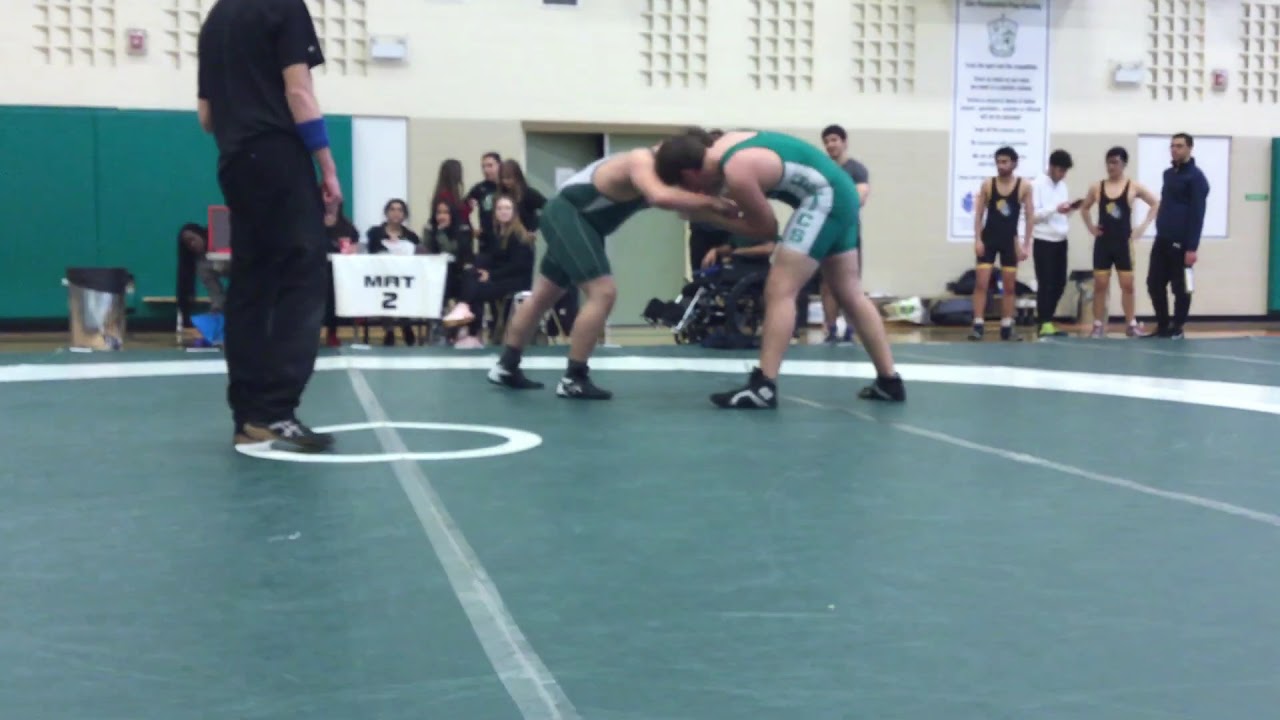In the foreground of the image, two Caucasian wrestlers in green uniforms with white trim are engaged in a match, locked together on a dark green mat that features white circles and lines. Both wrestlers are wearing black tennis or wrestling shoes. The wrestler on the left has the letters "C" and "S" visible on his uniform. To the right, a referee dressed in a black shirt, black slacks, and a blue wristband on his right arm is closely observing the match. Surrounding the mat are numerous spectators; some are standing, others sitting, and a group of ladies are seated at a table draped with a white cloth bearing the letters "MRT" in black. The background features a wall that transitions from white to green to cream, with a white poster and a visible doorway. Other wrestlers in uniforms are also seen watching the match, intensifying the competitive atmosphere.